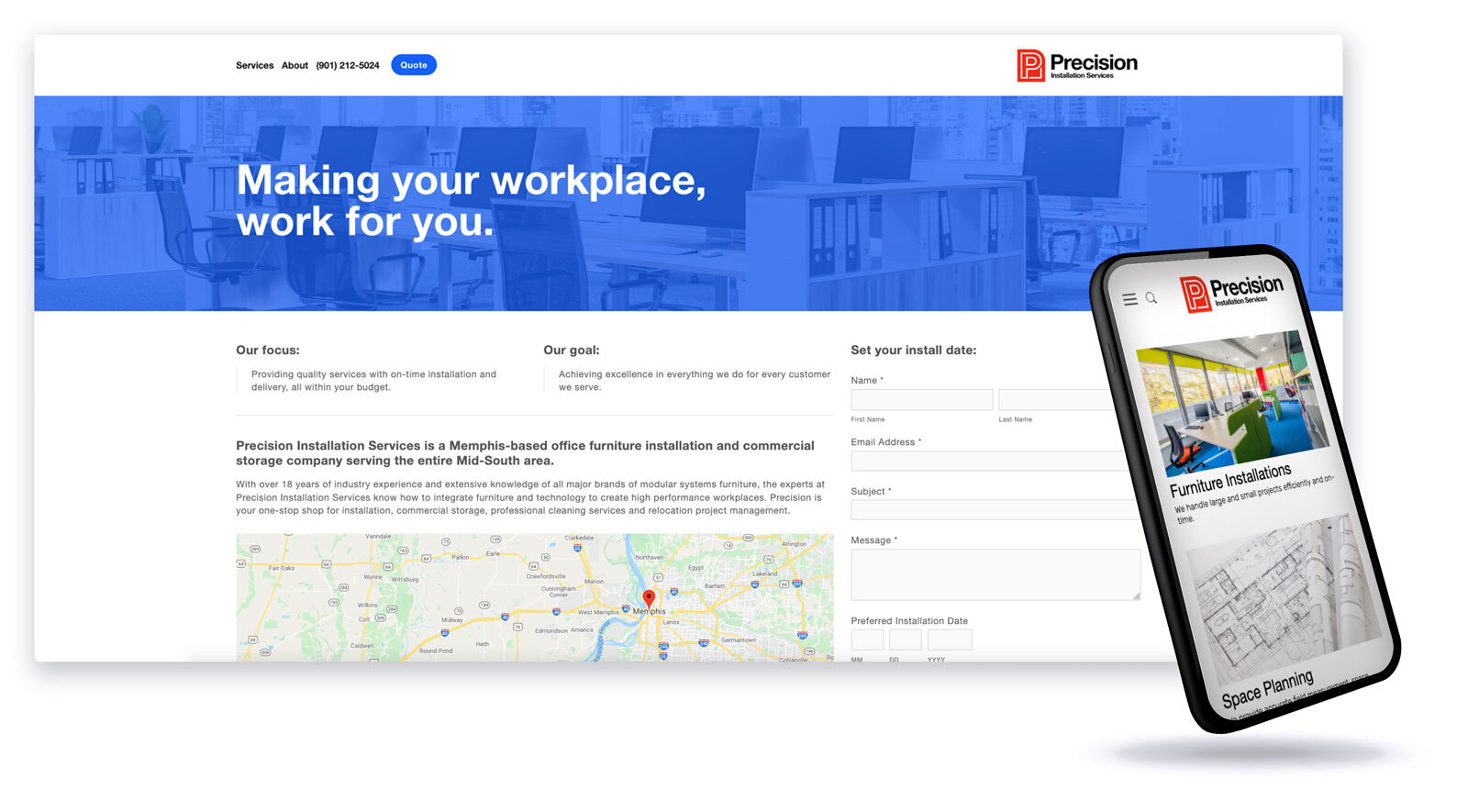In this image, we see a detailed screenshot of a web page, featuring a variety of elements that provide insight into the business being showcased. 

**Top Right Corner:**  
A distinctive logo for "Precision Installation Services" is prominently displayed, establishing the brand identity.

**Header Section:**  
A striking blue header adorns the top of the page, featuring an image that showcases a professional workspace. The image includes office equipment such as a desk, chairs, and computer screens, conveying a modern and efficient office environment.

**Primary Content Area:**  
Beneath the header, the page provides a thorough explanation of the business. The text begins with key points highlighting their focus and goal: 
- **Focus:** Providing quality services with on-time installation and delivery, all within the customer's budget.
- **Goal:** Achieving excellence in every endeavor for every customer served.

An extensive paragraph further elaborates on the company's identity and expertise:
- **Company Overview:** "Precision Installation Services is a Memphis-based office furniture installation and commercial storage company serving the entire Mid-South area."
- **Experience and Knowledge:** With over 18 years of industry experience and a profound understanding of all major brands of modular systems furniture, the experts at Precision Installation Services excel at integrating furniture and technology to create high-performance workspaces.
- **Comprehensive Services:** The company is described as a "one-stop shop," offering services that include installation, commercial storage, professional cleaning services, and relocation project management, catering to a wide range of customer needs.

**Right-Side Section:**  
On the right side of the page, there is a functional interactive element, an option to "Set Install Date." This feature allows users to enter their personal information, presumably to schedule an installation date, enhancing user engagement and providing a practical service directly through the webpage.

Overall, the webpage is thoughtfully laid out to highlight the company's capabilities, experience, and customer-centric focus, inviting potential clients to engage with their services easily and efficiently.